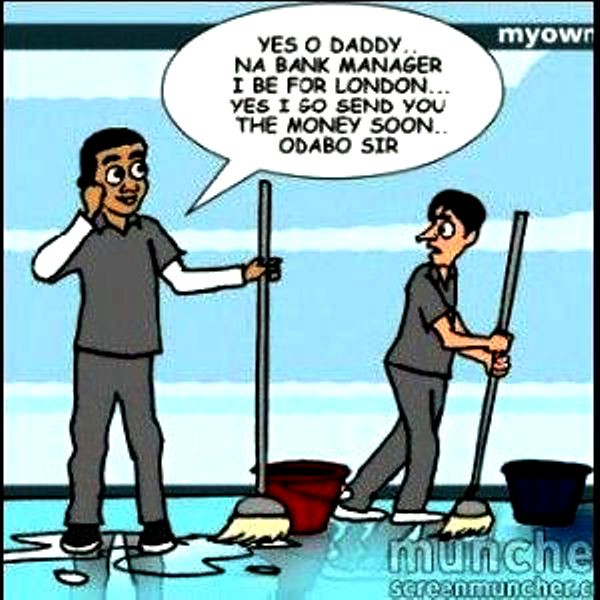The comic strip depicts two cartoon janitors standing next to each other on a shiny blue floor, in front of a large glass window that shows a blue sky with long, horizontal white clouds. Both men are wearing gray janitor uniforms — gray collared tops, gray pants, and their respective shoes: white for the Caucasian man on the right and black for the black man on the left. Each man holds a mop with a gray pole and a white brush. The black janitor, standing in a puddle next to a red bucket, has his right hand up to his face while talking on the phone. He is mid-conversation with a speech bubble reading, "Yes, oh daddy. Nay bank manager. I be for London. Yes, I go send you the money soon. Adabo, sir." The white janitor, positioned next to a blue bucket, looks at his colleague with a frightened expression. The comic has a watermark at the bottom right corner, stating "Munch, ScreenMuncher.com."